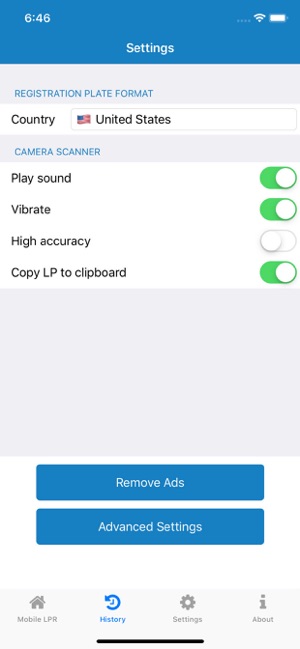The image showcases a settings screen on a mobile device, detailing at 6:46 AM with full signal strength (indicated by four filled dots), active Wi-Fi, and a fully charged battery at 100%. All these indicators, alongside the word "Settings," are displayed in white on a blue bar at the top.

Beneath this blue bar is a gray rectangle with "Registration Plate Format" written in blue. This is followed by a white text box containing the pre-filled text "Country" and an American flag, representing the United States.

Next, there is another gray rectangle with "Camera Scanner" written in the same blue color. Below this are several white spaces featuring toggle buttons for different options: "Play Sound" (on), "Vibrate" (on), "High Accuracy" (off), and "Copy LP to Clipboard" (on).

Further down, a large gray space devoid of text separates the toggles from two blue buttons with muted white text that read "Remove Ads" and "Advanced Settings." Another gray bar appears at the bottom of the screen.

At the very bottom, a menu displays options: "Mobile LPR" (with a house icon), "History," "Settings" (mimicking a gear/cog icon and highlighted in blue, indicating focus), and "About" (with an 'i' icon). All the options, except for "Settings," are in gray, delineated by a black line beneath them.